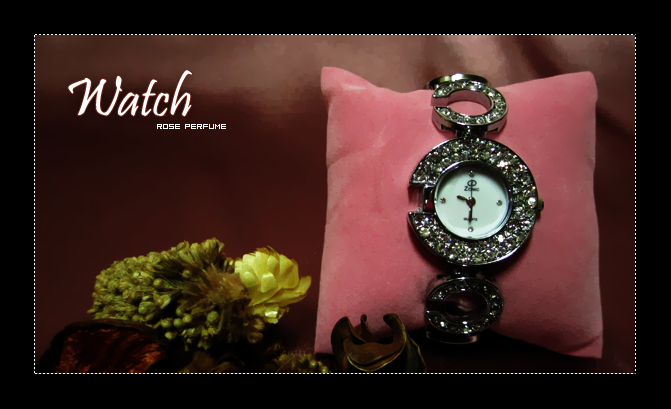This advertisement features a luxurious watch displayed within a black rectangular border adorned by a perforated line of white dots. In the top left corner, the text "Watch Rose Perfume" is elegantly written in white, with 'Watch' in a fancy script and 'Rose Perfume' in more straightforward block letters. The background of the ad has a rich brownish-purple hue. Situated at the bottom left corner is a small green plant, next to which stands a yellow flower. 

To the right, the watch, encrusted with what appears to be either diamonds or cubic zirconias, is elegantly wrapped around a pink velvet pillow. The wristwatch showcases a silver design with the face of the clock in light blue or white, displaying the time as 9:30. The watch, although featuring a brand that starts with the letter "Z," has brand details that are obscured. This luxurious piece, with its intricate detailing, stands out against the slightly blurry background items, making it the focal point of the ad.